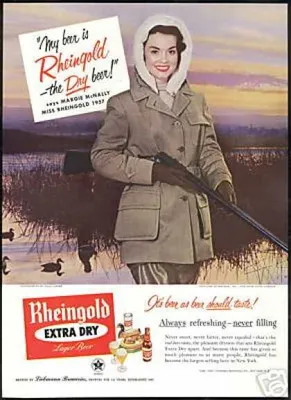The vintage promotional poster features a cheerful woman, dressed warmly in a khaki winter coat with a hood, standing in a natural setting resembling a duck hunting scene. With brown leather gloves, she holds a break-action, double-barrel shotgun pointed safely to the right, its barrel open to indicate a non-aggressive stance. Behind her is a scenic pond with ducks and tall grass, under a picturesque early morning sky flushed with pink, purple, and yellow hues. Text on the upper left corner reads, "My beer is Rheingold the Dry Beer," while additional text, "Always refreshing, never filling," emphasizes the brand’s slogan. The bottom half of the poster features the Rheingold Extra Dry logo on a large white background, along with illustrations of beer steins and bottles, reinforcing the vintage mid-20th-century aesthetic. This advertisement clearly targets a market of outdoor enthusiasts, aiming to associate the beer with refreshing and never filling qualities.